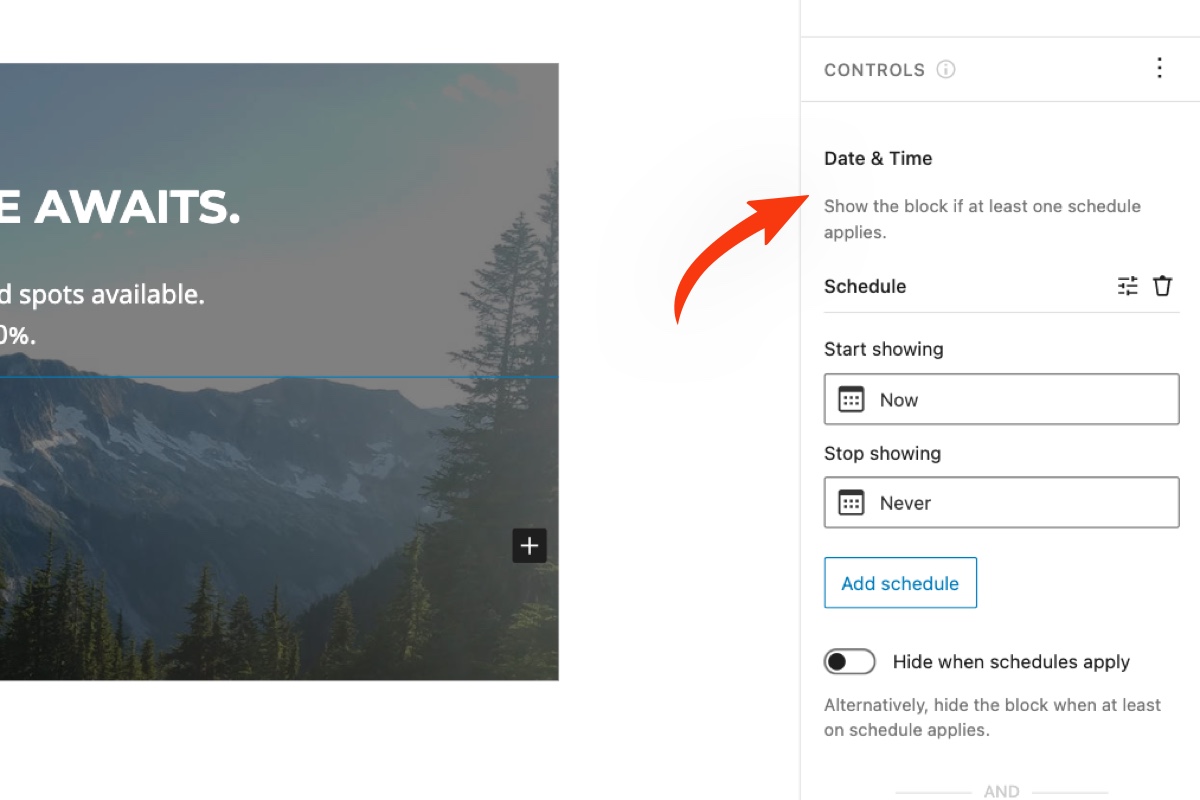The image is split into two sections. On the left-hand side, the image is partially cropped, displaying text with a bold white letter "E" that is cut off and unreadable, followed by the word "awaits" and the phrase "spots available" beneath it. The background features evergreen trees at the bottom, brown mountains in the distance with patches of white snow, and an overcast sky above.

Adjacent to this, a red arrow has been digitally added, pointing towards the right-hand side where detailed information about "date and time" settings is shown. Above this, the word "controls" can be seen. Further descriptions include "Show the block if at least one schedule applies," alongside a filter icon indicating "schedule showing now, stop showing never." Options for "Add schedule" and "Hide when schedules apply" are also visible, with additional instructions for hiding the block when at least one schedule is active.